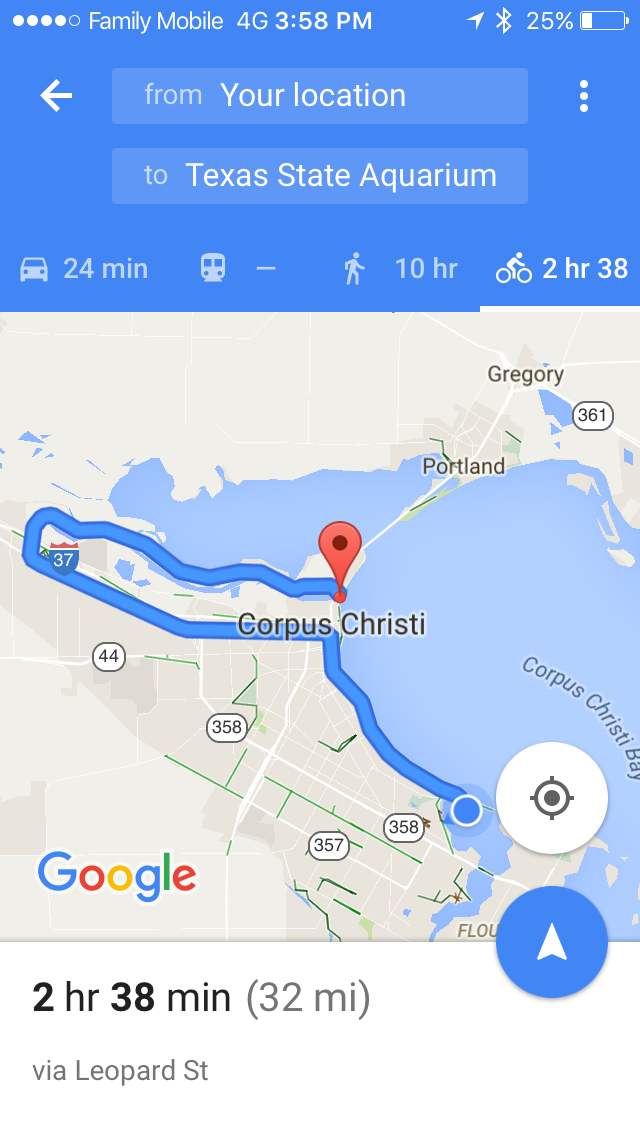A Google Maps image displays detailed bike directions from an unspecified starting location to the Texas State Aquarium. It highlights various transportation modes represented by symbols: a car, a train, a walking person, and a bicycle. The bike route, which covers a 32-mile distance, is estimated to take 2 hours and 38 minutes. Car travel to the destination is noted to be a 24-minute drive, no ETA is given for train travel, and walking would take approximately 10 hours.

The map also features several roadways with labeled numbers such as 358, 357, and 44, although these are adjacent to but not part of the selected route. The main travel path follows along Interstate 37. Key landmarks include a red pin marking the destination at the Texas State Aquarium and a blue dot indicating the starting point. Additionally, the map highlights Corpus Christi Bay with a blue patch, emphasizing its proximity to the route.